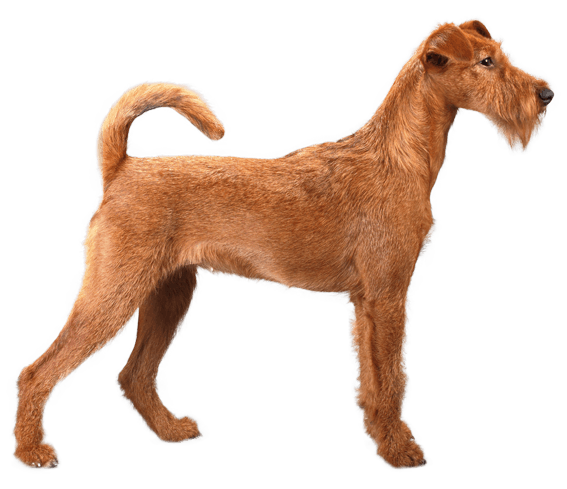The photograph features a medium-sized, brownish-tan dog with a reddish hue, closely resembling an Irish Terrier or a mix with a Scottie. This canine stands upright and alert on a white or transparent background, fully occupying the frame. It faces to the right, showcasing its side profile. The dog has distinct floppy ears that fold forward and a slightly elongated snout adorned with a wispy beard-like tuft of hair. Its dark, intelligent eyes give it a watchful and calm demeanor. The dog exhibits a sturdy build, with long legs positioned to display a sense of readiness—its left back leg slightly ahead of the right, while the front legs are symmetrically aligned. The tail is notably short and curls back towards its body, resembling an upside-down "U." The overall impression of the dog is that of attentiveness, as if it's observing something in the distance. No background elements are visible, emphasizing the dog's presence in the image.